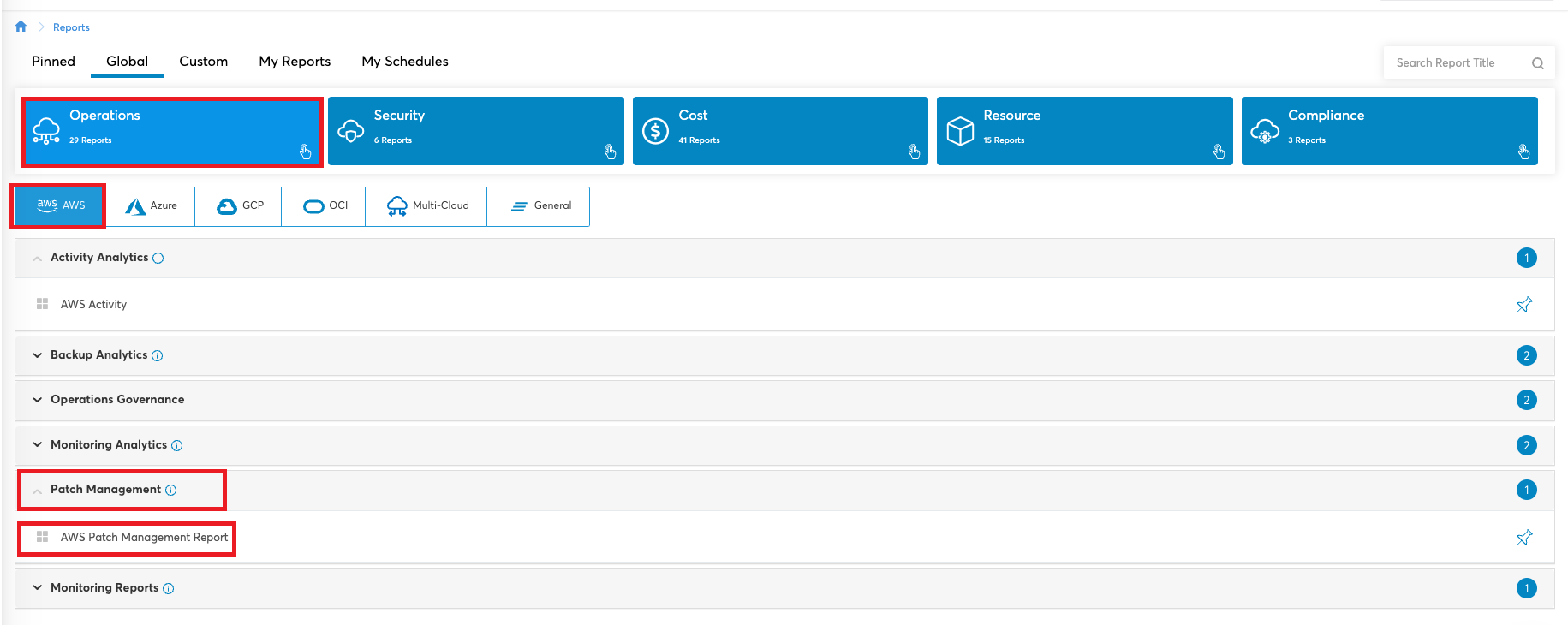Here is a cleaned-up and detailed caption for the image described:

"The screenshot captures the Amazon Web Services (AWS) dashboard interface, showcasing various menu elements and options. At the top of the screen, the home button is visible with the 'Reports' section expanded. Below this, there are multiple categories listed: Pinned, Global, Custom, My Reports, and My Schedules. The 'Global' category is underlined, indicating it is currently selected. Within this category, the dashboard displays several report types along with their respective counts: Operations (29 reports), Security (6 reports), Cost (41 reports), Resource (15 reports), and Compliance (3 reports).

The interface includes a search bar labeled 'Search Report Title' for easy navigation. The 'AWS Operations' section, highlighted in a red box, shows 29 reports. Additionally, the screen offers options for other cloud services such as Azure, GCP (Google Cloud Platform), OCI (Oracle Cloud Infrastructure), Multi-cloud, and General.

The selected report focuses on 'AWS Patch Management,' marked by a red box. Below it, various activity analytics categories are listed including AWS Activity, Backup Analytics, Operational Governance, and Monitoring Analytics. The 'Patch Management' report, also highlighted in red, is titled 'AWS Patch Management Report' and falls under the 'Monitoring Reports' section, which has been pinned for quick access."